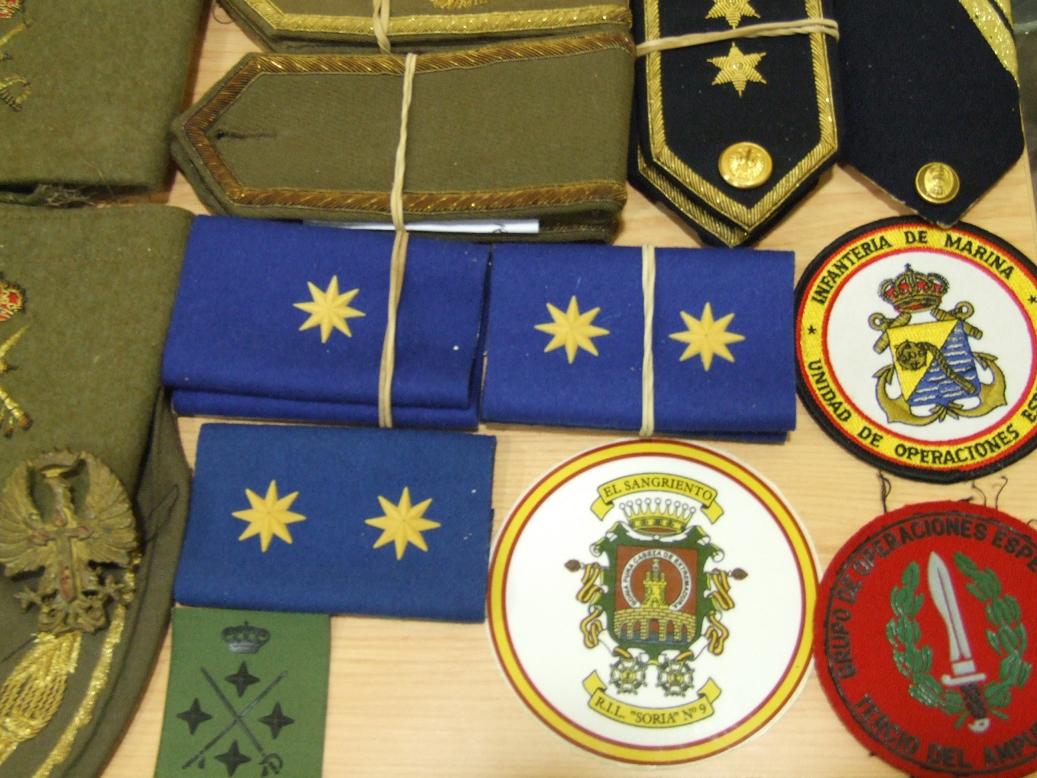This photograph features a diverse collection of military service patches, rank insignia, and embroidered lapel accessories that are typically worn on military uniforms. The majority of the patches have Latin-based language inscriptions. Central to the display is a circular patch labeled "Infantería de Marina, Marine Infantry, Unidad de Operaciones," with additional wording that is partially obscured. 

The collection includes various shapes of patches, such as circular, rectangular, and epaulette straps. Among these, a notable detail is a set of blue patches adorned with eight-pointed gold stars. To the left side of the image, some patches are dark green, with one displaying a crown and four black stars. Several items feature intricate designs, such as a yellow-bordered patch with a red rim and a complex gold-fringed insignia at the top.

One circular patch towards the bottom right is red with black letters encircling a central image of a knife surrounded by a wreath. Another prominent patch nearby is bordered in yellow, edged by red on either side, featuring a shield with multiple designs flanked by the phrases "En Sangrito" and "R.I.L. Soria No. 9" on gold banners. These elements are indicative of the honored ranks and units these patches represent.

Grouped with rubber bands, these patches may signify someone’s military service achievements or could be displayed for sale. This collection vividly portrays the rich history and detailed craftsmanship emblematic of military uniforms and insignia.